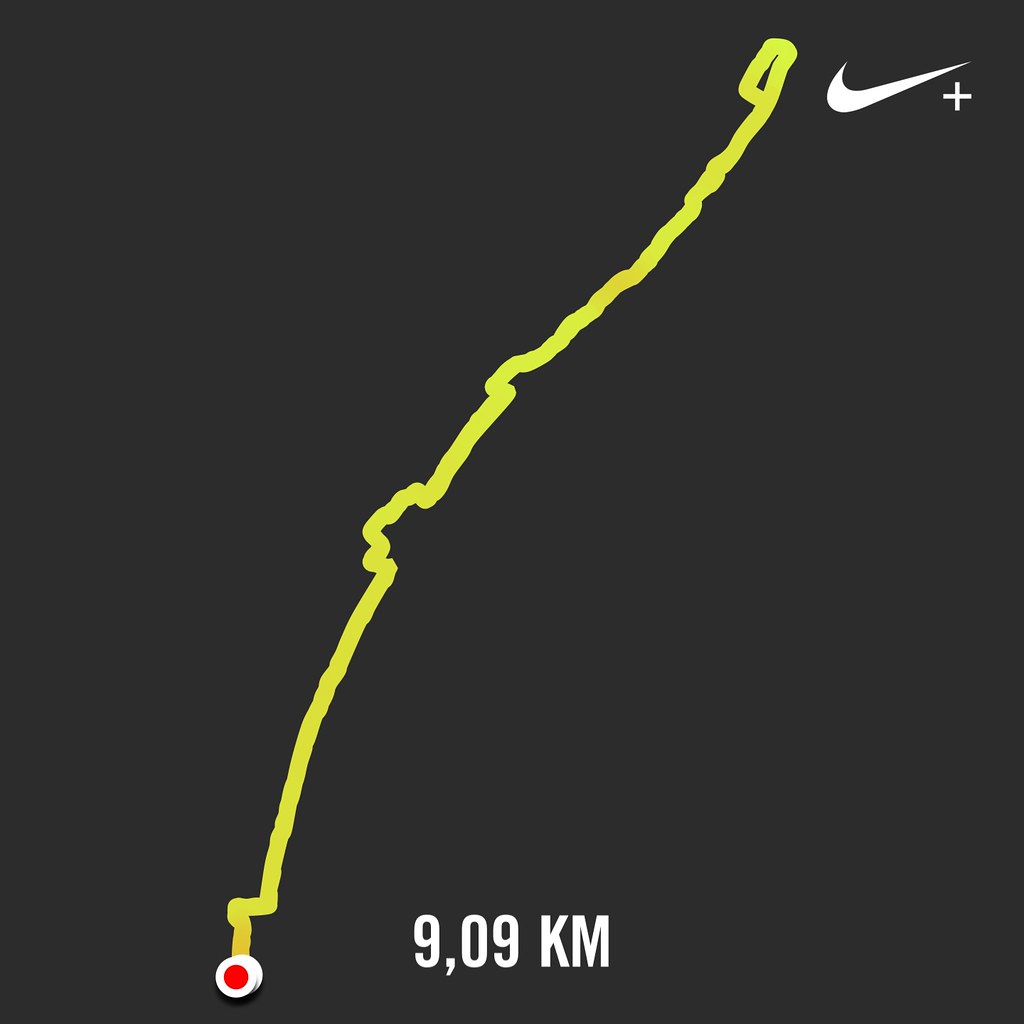The image features a minimalist design with a completely black or dark gray background. Prominently displayed in the top right corner is the white Nike logo accompanied by a small plus sign. Cutting diagonally across the image from the bottom left to the top right is a thick, neon yellow squiggly line. This dynamic line, which resembles a very basic and jagged path or map, starts at a white pin with a red center located at the bottom left of the image. It moves upwards in a non-linear fashion, featuring multiple curves and humps, before reaching its end. Below the starting pin, in bold white capital letters, the text "9,09 KM" is clearly visible, indicating a distance of 9.09 kilometers. The overall design is simplistic and vector-like, focusing on these central elements without any additional details or alterations.